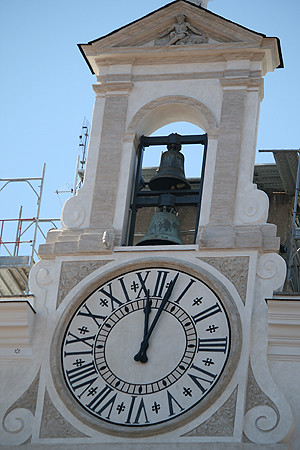The photograph showcases an impressive, possibly government, building with a distinct architectural design. The structure features a prominent marble clock tower that narrows to a pointed top. The clock face, large and white, displays the time as 12 o'clock, suggesting it is noon given the bright blue sky. Above the clock are two weathered bronze bells, now green from exposure to the elements, housed within a post-and-lintel structure beneath a triangular pediment. Inside this pediment, there is a detailed sculptural figure. Surrounding the clock are elegant curves and waves, giving the facade a sophisticated finish. In the background, there is visible construction activity, including scaffolding and eaves. Despite the traditional Greek and Roman architectural influences, the tower's pristine appearance hints that it is either well-preserved or a recent addition designed to evoke classical aesthetics.